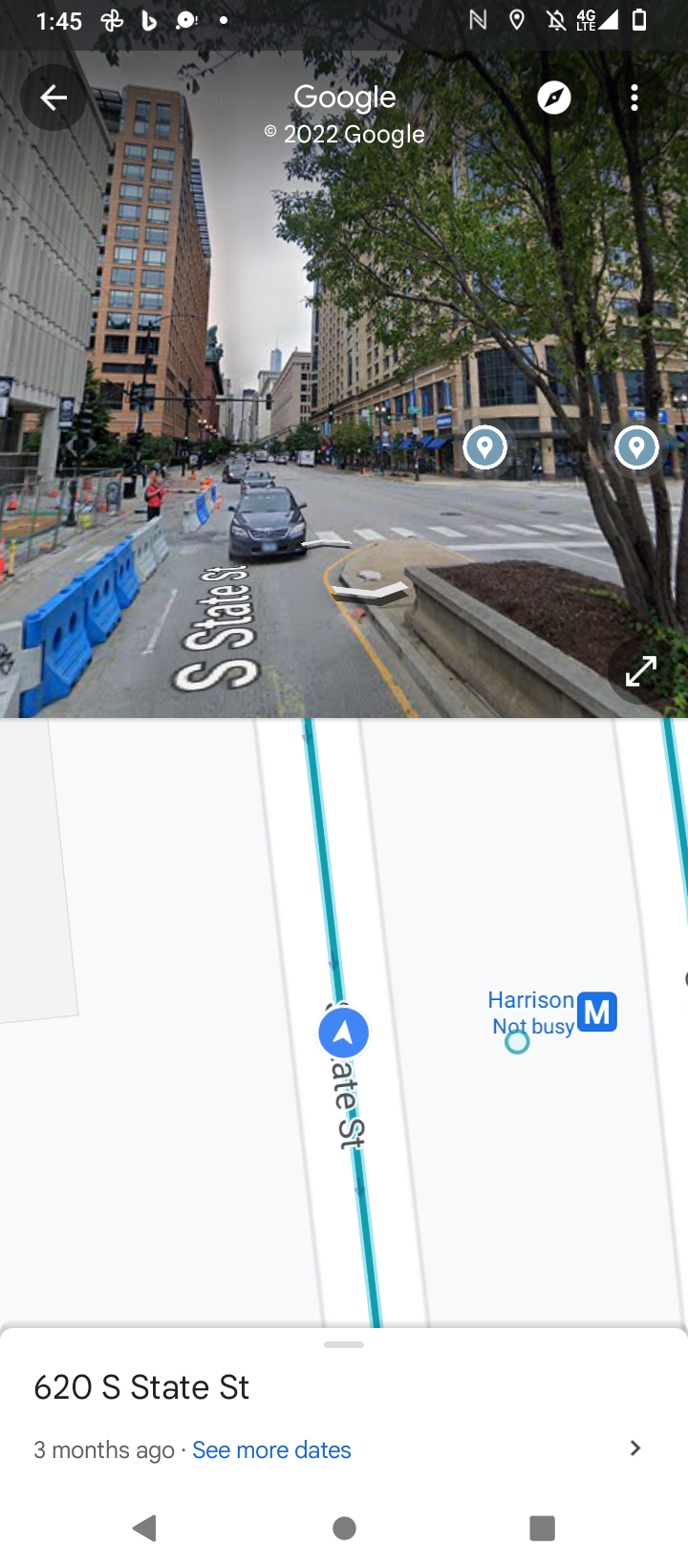A detailed caption for this image could be:

"This screenshot captures a phone displaying the Google Maps app. The top half of the screen features a Street View image of South State Street, showcasing several buildings, a car approaching the viewer, and pedestrians walking along the sidewalk. A tree can also be seen in the scene. The vertical text 'South State Street' is accompanied by forward and backward navigational arrows. The top of the screen includes the Google Maps interface, with 'Google 2022 Google' displayed prominently. The phone's taskbar at the very top shows the time as 1:45 PM, along with various app notifications and the battery level indicator. The lower half of the screen presents a traditional map view, where a blue line traces State Street. To the right, there is information indicating that Harrison is 'not busy' along with an 'M' icon. At the bottom of the screen, the text '620 South State Street' appears, along with a note that this location was viewed 'three months ago' and an option to 'see more dates.' The phone's navigation bar displays icons for the home screen, back, and recent apps functions."